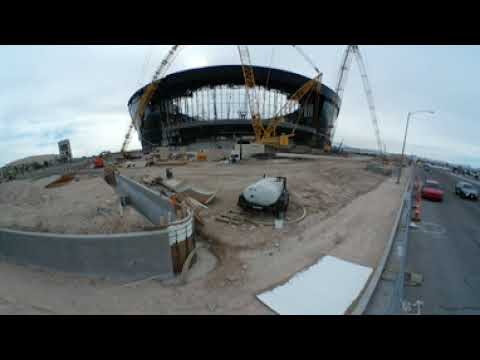The image depicts a bustling construction site at the center of the frame, dominated by a large, bowl-shaped stadium. Surrounding the stadium are several towering yellow cranes with numerous cables hanging from them, contributing to the complex construction activity. The ground around the stadium and throughout the construction site is primarily light brown dirt, indicative of significant land clearing. A prominent concrete barrier runs along the left side of the image. On the right side, a road stretches along the edge, with a red car and a dark grey car visible on it, and a streetlight positioned halfway down the sidewalk.

The sky above is partly cloudy, adding depth to the outdoor scene, which appears to be captured in the middle of the day. 

A black border frames the image, and a hint of greenery can be seen on a small hill to the far left, with more populated settings visible along the bottom and far right. Various construction vehicles and equipment, including what appears to be a tank possibly used for water storage, are scattered around the stadium. The context is enriched by the contrast between the dry soil of the construction area and the complex structure of the stadium being built. There is no text present anywhere in the image, and the color palette includes black, tan, white, red, yellow, orange, brown, and gray.